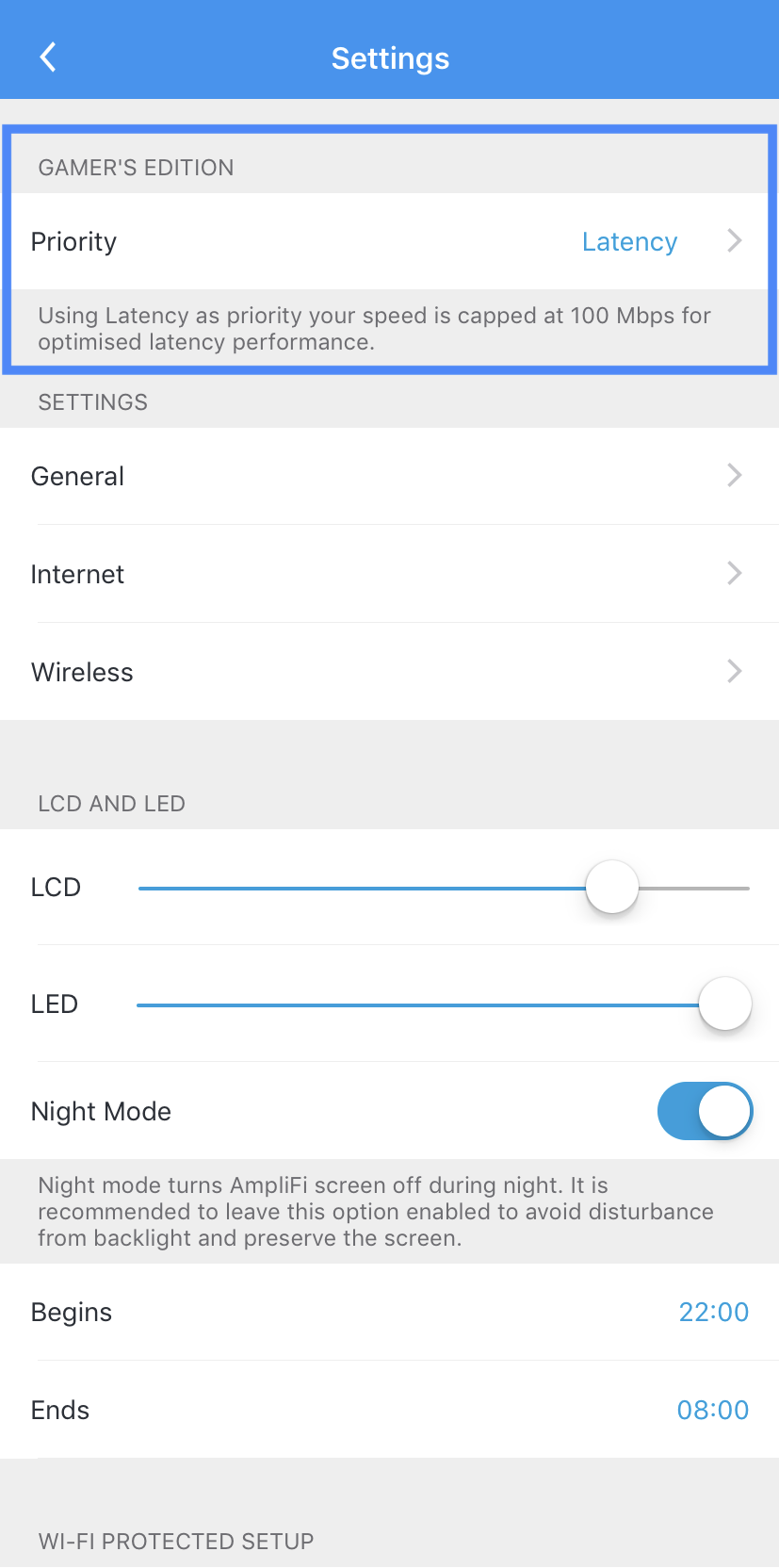This image displays the settings page of a smartphone, with a greyish and white background. At the top, a blue bar prominently reads "Settings," followed by the section title "Gamers Edition" outlined in blue. Under "Gamers Edition," an option labeled "Priority" appears, with "Latency" to the right. Users can select their latency settings by clicking on this option. A note below in small text explains, "Using Latency as Priority. Your speed is capped at 100 Mbps for optimized latency performance."

The next section, "Settings," presents three options on a white background: "General," "Internet," and "Wireless." Following this is the "LCD and LED" section, containing three more options: "LCD," "LED," and "Night Mode." These options feature adjustable bars for user interaction. The "Night Mode" option is toggled on, with a note beneath it stating, "Night Mode turns Amplify screen off during the night. It is recommended to leave this option enabled to avoid disturbance from backlight and preserve the screen." Additionally, beneath this are "Begins" and "End" settings to specify the start and end times for Night Mode.

The final section pertains to "Wi-Fi Protected Setup," but no further information is visible under this heading.